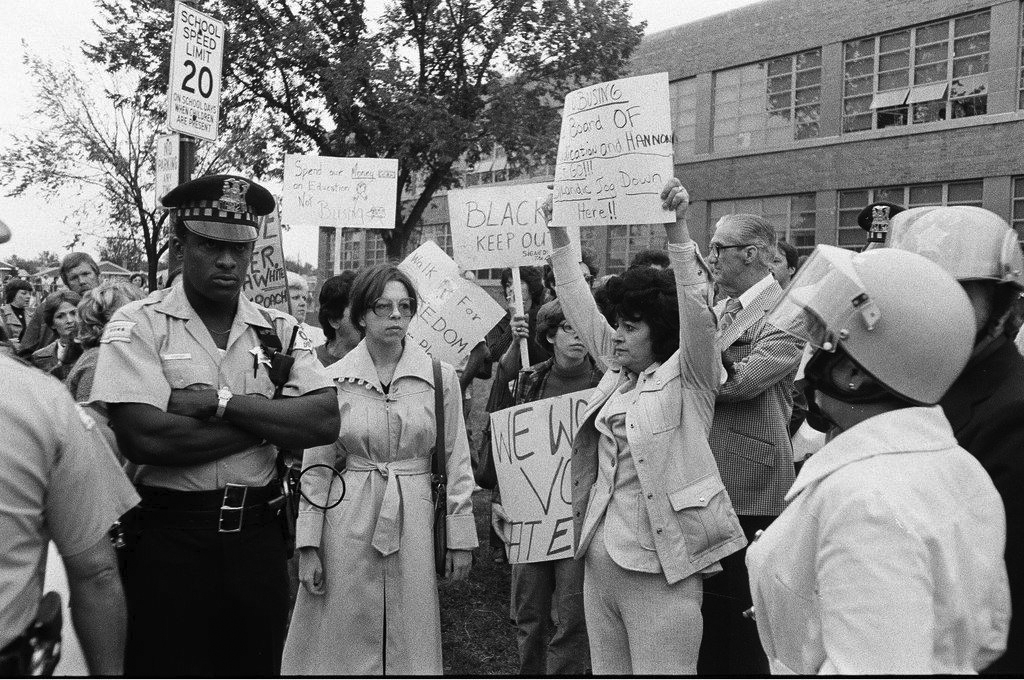The black-and-white photograph, likely from the 1960s, is a powerful and evocative depiction of a protest outside a public school. The two-story building in the background, located in the top right corner, features large multi-pane windows, some of which are open to let air in. The crowd, occupying the bottom half of the image and stretching from the left to the right side, is composed of a diverse group of individuals holding large white signs with various messages, including some that read "Black Keep Out" and "Abusing Board of Registration."

At the center of the image stands a prominently featured woman with afro hair, wearing trousers, a jacket, and a smaller suit jacket underneath. She raises a placard above her head, adding to the visual intensity of the scene. Scattered throughout the crowd are several uniformed police officers. Some wear riot helmets with visors, while others don traditional police caps with crests. Notably, an African-American police officer is at the center, assumed to be monitoring the situation, which seems tense and poised for aggression.

Adding to the atmosphere, there are sparse trees visible in the background behind the building, anchoring the scene in a typical urban setting from the era. The photograph captures a moment rich with historical significance and emotional weight as people protest against racial integration in the school system.